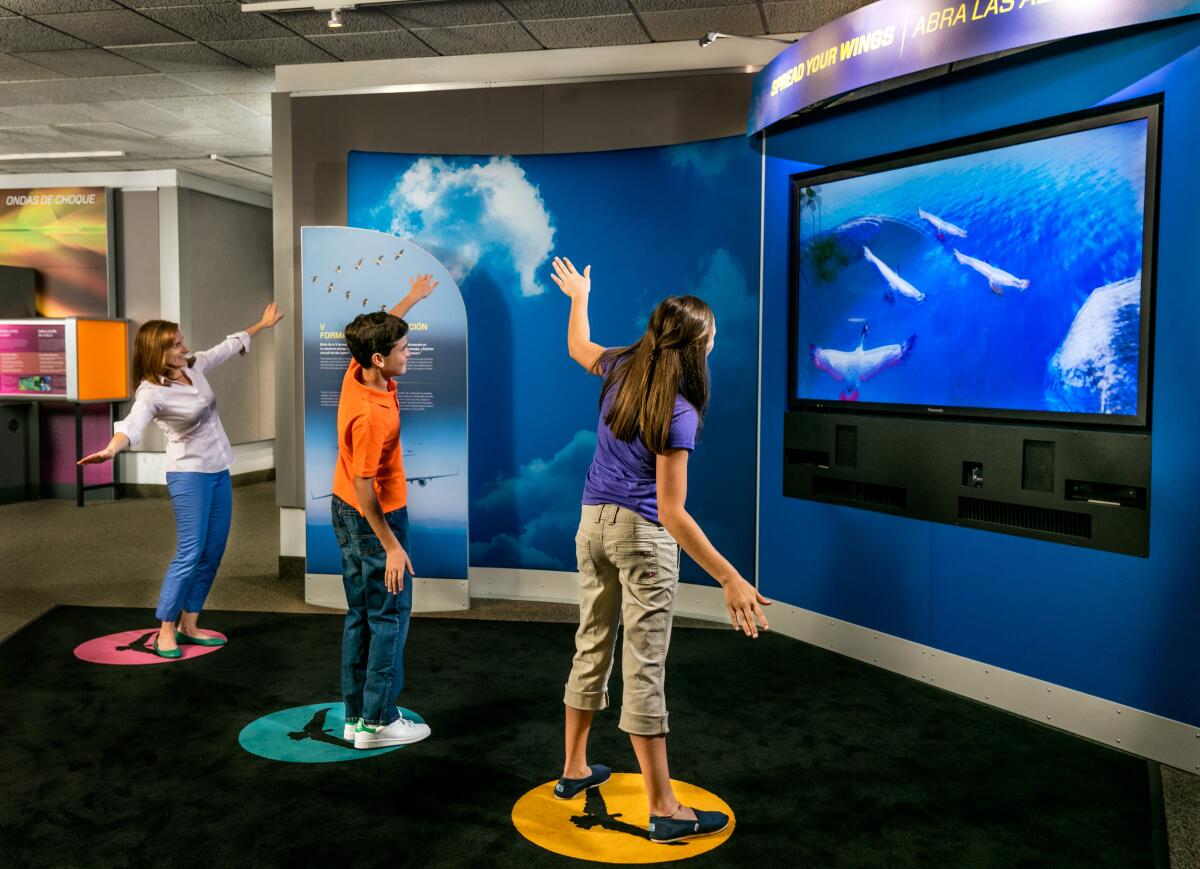In this vibrant photograph, three individuals—an adult woman and two children—are engaged in an interactive exhibit at a museum. They are positioned on brightly colored pads that are part of a bird simulatory experience. The woman, wearing a purple shirt, stands on a pink pad, the boy in an orange shirt and jeans on a blue pad, and the girl in a white shirt and blue pants on a yellow pad. Their arms are stretched out, mimicking the flapping of wings as they immerse themselves in the experience. Mounted on the blue wall in front of them is a large TV screen displaying birds flying over water, seemingly controlled by the movements of the participants. Above the screen, the caption "Spread Your Wings" is prominently displayed, alongside partial Spanish text "Abra las...". The left side of the wall features another image, likely showcasing clouds. The scene hints at a rich, educational environment, possibly with additional informational panels referencing geese in flight and other interactive elements scattered throughout the museum space.